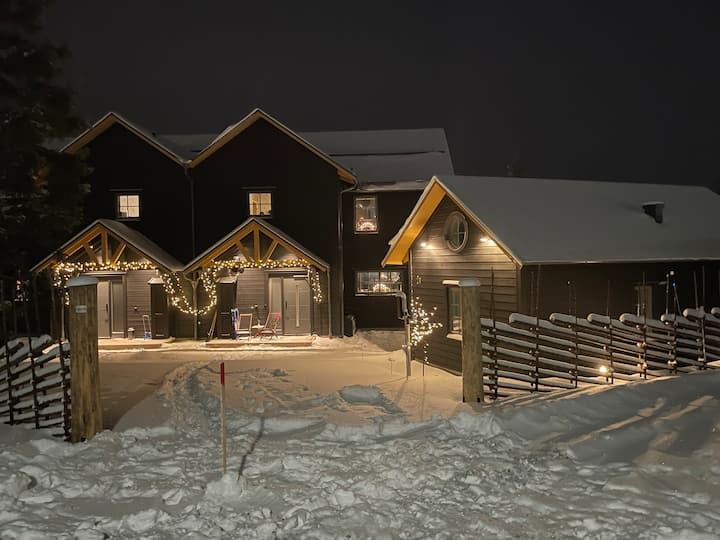This captivating nighttime photograph showcases a cozy winter scene framed by softly glowing Christmas lights. The landscape, blanketed in a fresh, textured layer of snow, features two charming wooden townhouses. Each house, painted a warm brown and topped with A-frame roofs, stands nestled within a fenced-in yard. The structures boast multiple front doors, hinting at multi-family dwellings, and festively decorated porches. Twinkling holiday lights adorn the entrances, casting a muted, inviting glow, amplified by the gentle porch lighting. Footprints crisscross through the snow, carving winding paths to the front doors. A wooden fence, beginning in the lower left foreground, meanders across the scene, adding to the rustic charm. In the background, dark silhouettes of trees are barely visible against the inky sky, accentuating the serene ambiance of this winter wonderland. Subtle movements within the windows of the left-side building reveal a lively interior, contrasting with the tranquil, snow-covered exterior.